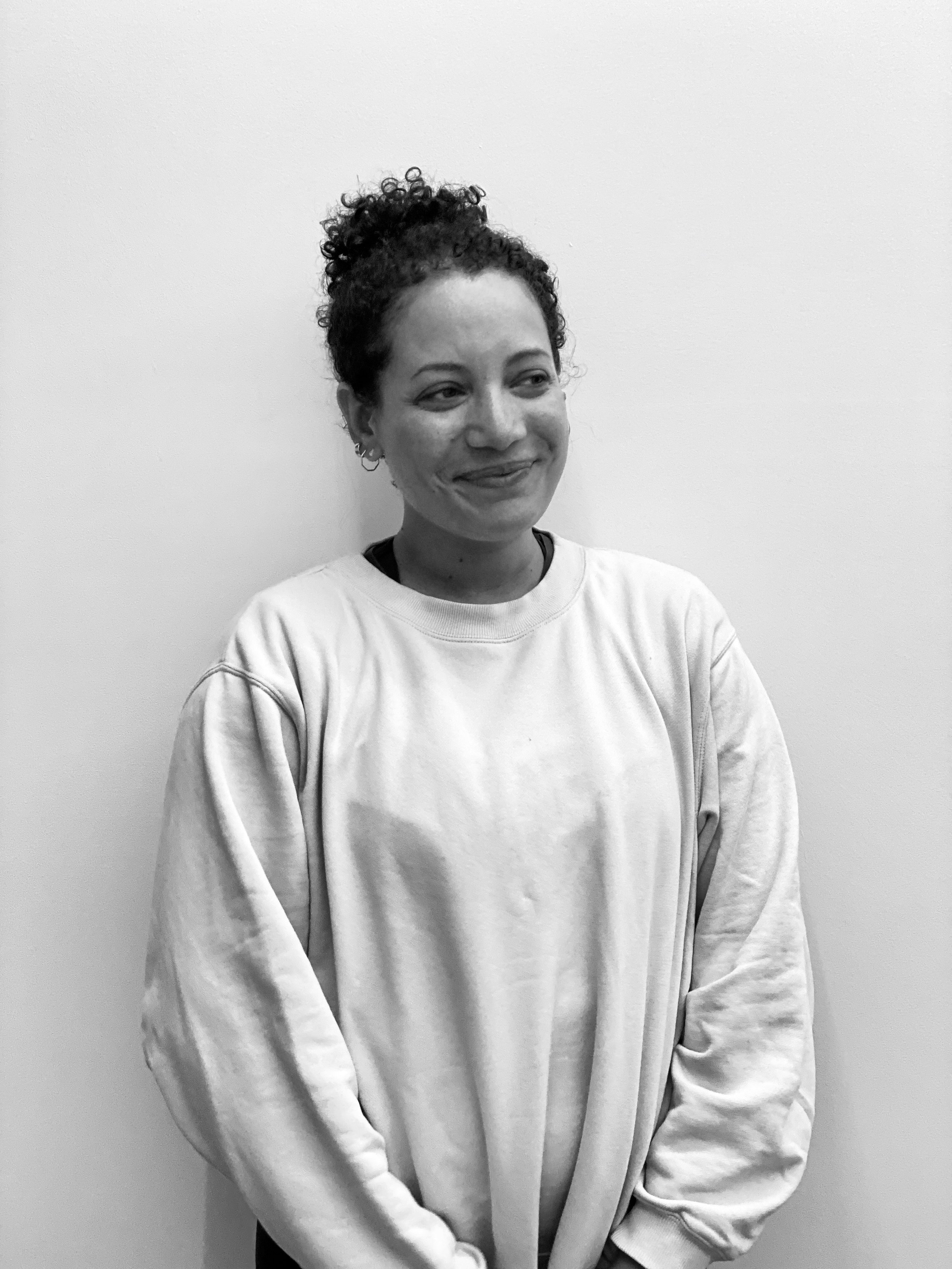This is a recent black and white photograph capturing a young woman, likely in her mid-20s to mid-30s, against a slightly gray wall without a border. The vertically rectangular image focuses on her upper body. She has short, very curly dark hair pulled up into a bun, revealing her right ear adorned with a small loop earring, while her left ear remains out of sight. The woman is dressed in a dark t-shirt layered under a long-sleeved, light-colored sweatshirt of a crew neck, slightly resembling a light sweater. Her expression is marked by a subtle, closed-mouth smile as she glances off to her left, adding a contemplative touch to her demeanor. Shadows cast from her figure are faintly visible on the wall behind her.